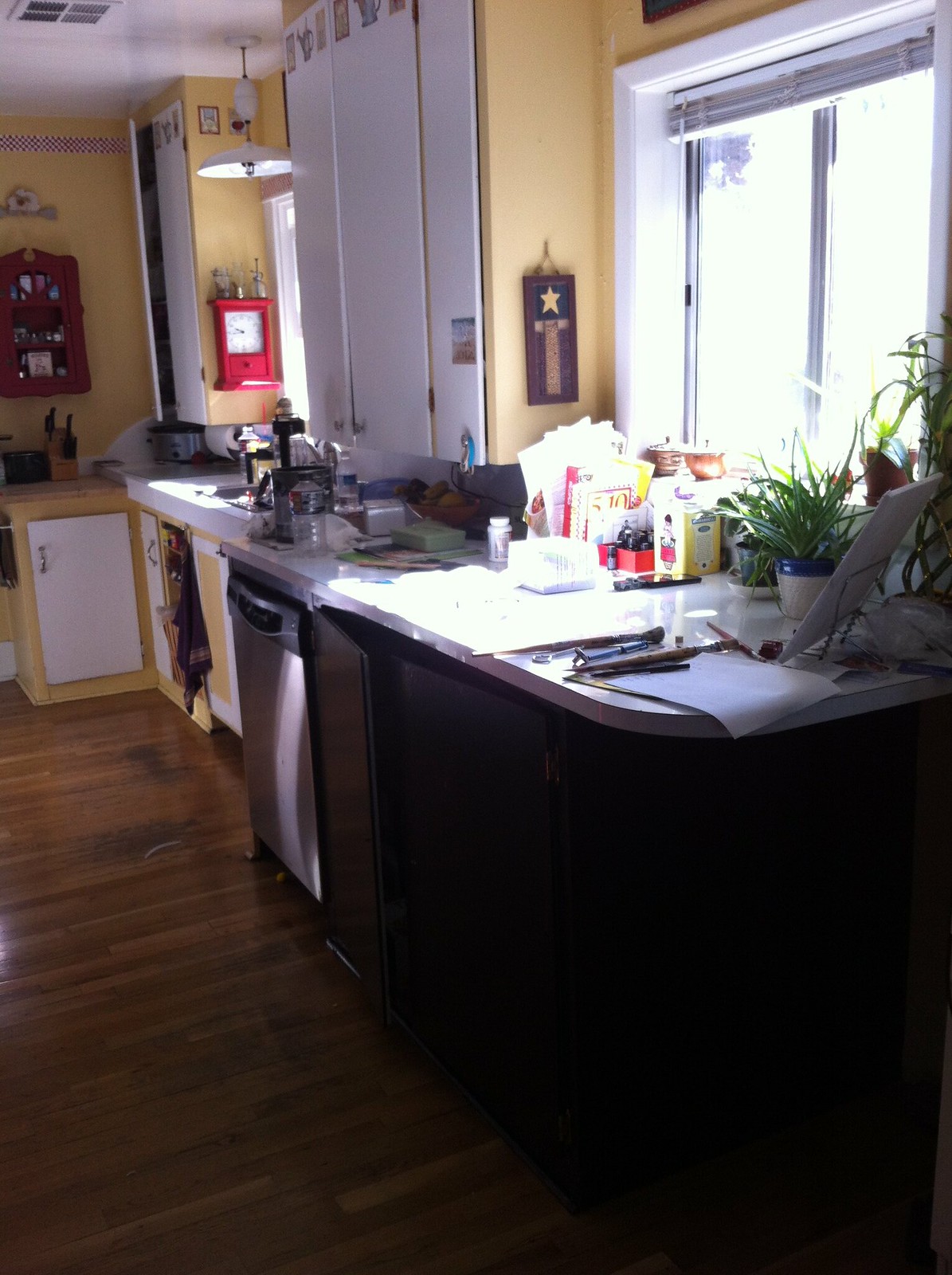This photograph depicts a cozy kitchen bathed in warm, yellow tones. The focal point is a long, wooden counter that extends to a sink at its end. Adjacent to the sink, nestled below the counter, is a sleek dishwasher. The counter stretches onward to a spacious area adorned with a window, where a tablet and some scattered papers occupy one corner. A small shelf above holds an assortment of books and more papers. The windowsill presents a charming array of jars or canisters, adding a touch of homely practicality to the scene. In the corner, a quaint wooden plaque hangs, adding a rustic charm to the setting. The cabinets in the foreground are crafted from wood, offering a striking contrast to the yellow and white cabinets in the background. The walls are painted a vibrant yellow, harmonizing with the overall decor. A red wall clock draws attention and provides a pop of color. In the background, a spice rack is conveniently positioned above a block of knives, indicating a well-equipped culinary space.